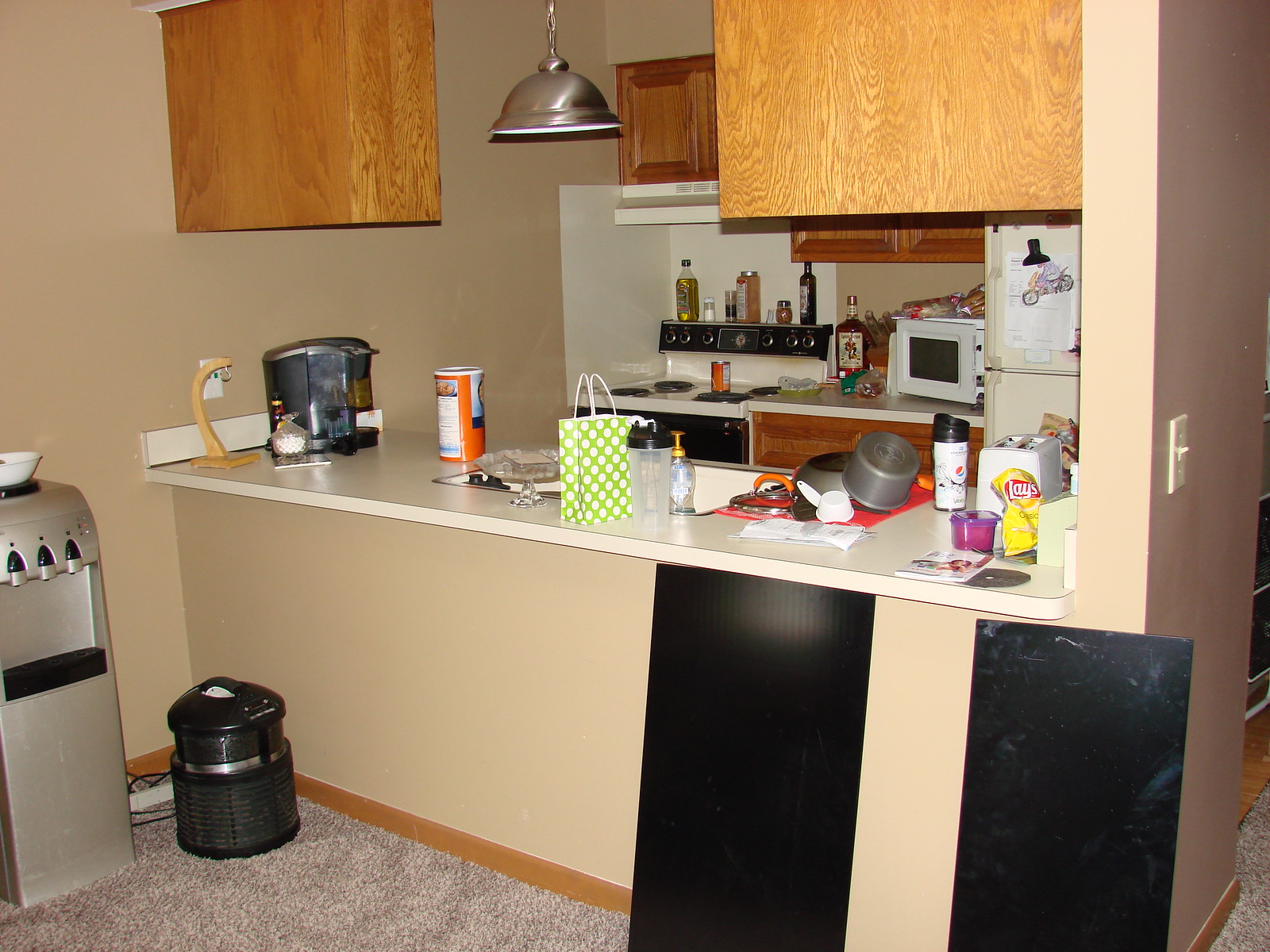The image captures the interior of an apartment, specifically focusing on the kitchen area as viewed from the adjacent living space. A bar counter with a partition wall serves as the boundary between the two areas. Leaning against this counter are two vertical black planks. In front of the bar, on the left, sits a silver rectangular water machine, and next to it on the floor is a black device, possibly a humidifier. Both are placed on a clean, cream-tan colored carpet.

The bar itself is a yellowy-cream color with a contrasting white countertop that is cluttered with various items. From left to right, the items include a wooden banana holder devoid of bananas, a Keurig coffee maker, and a small jar likely containing sugar. Centrally located is a container of oats next to a sink filled with items. Adjacent to the sink is a green and white polka-dotted gift bag, a shaker bottle, hand soap, and a stack of drying dishes on a towel, accompanied by a thermos.

On the right side of the bar, there is a white toaster, a random bag of Lay's chips, and assorted containers mixed with miscellaneous papers. Behind the bar, the back of the kitchen showcases an electric stove with a can resting on it, and the stovetop crowded with a bottle of olive oil, balsamic vinegar, salt, pepper, and other cooking essentials. To the right of the stove is a bottle of Captain Morgan rum, with more scattered items on the surrounding counters. A microwave is tucked into the corner, its top occupied by additional objects. The kitchen is enveloped by oak cabinets, and a silver light fixture hangs from the ceiling, illuminating the space.